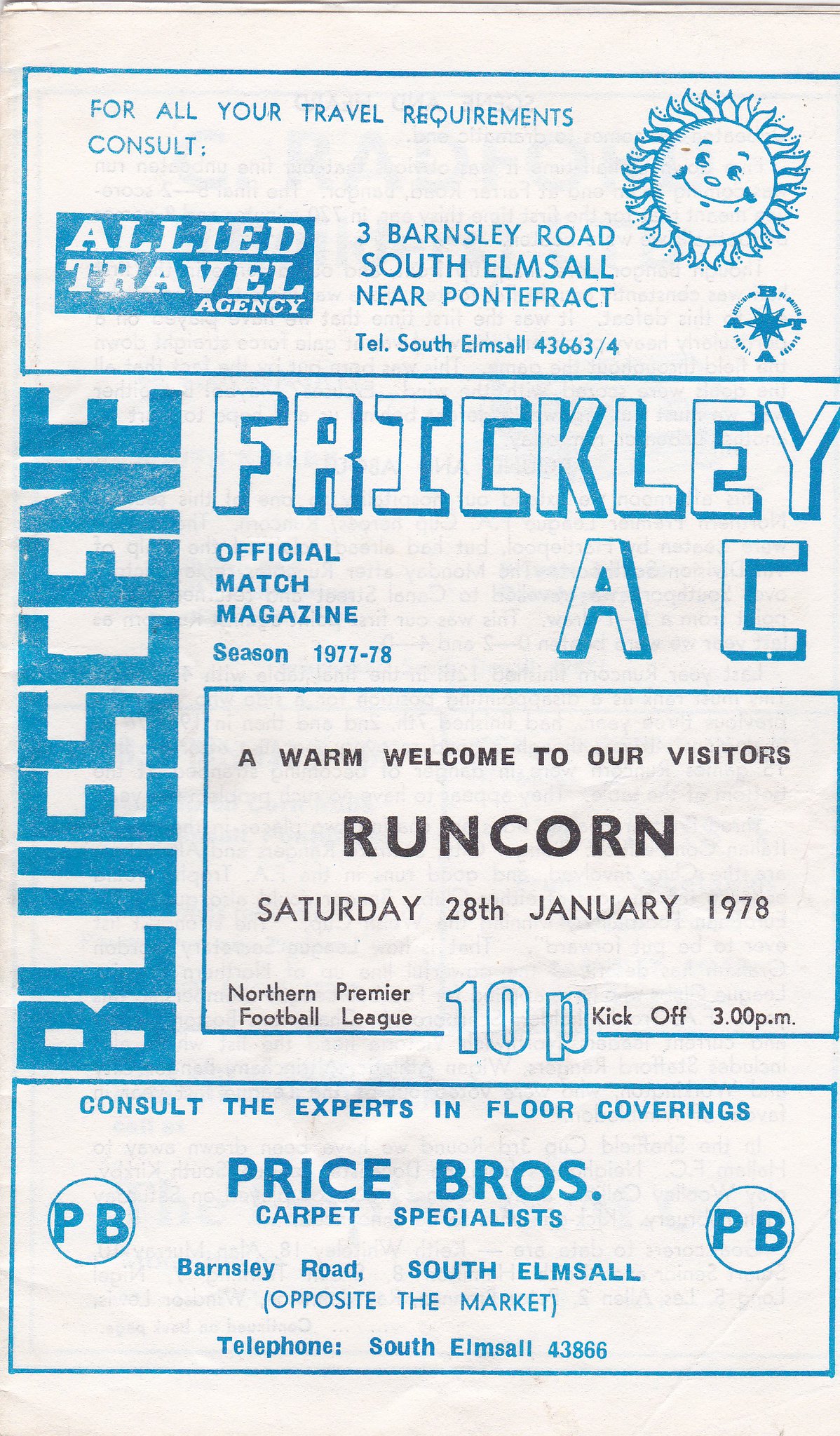The image displays a white magazine page from 1977-78, featuring predominantly blue text and a series of stacked advertisements. The top part of the page is an ad for Allied Travel Agency, stating, "For all your travel requirements, consult Allied Travel Agency." It provides the address, "3 Barnsley Road, South Elmsall, near Pontefract," and the contact number, "South Elmsall 43663-4." This is accompanied by a cheerful, grinning sun illustration. Below this, the page features the title "Blue Scene" in vertical text and identifies the publication as "Frickley A.C. Official Match Magazine, Season 1977-78." There is a section welcoming visitors from Runcorn for a match on "Saturday, 28th January 1978," part of the Northern Premier Football League, with a kickoff time at 3 PM. The bottom of the page contains another advertisement, urging readers to "Consult the experts in floor coverings, Price Bros, Carpet Specialists," located on "Barnsley Road, South Elmsall," opposite the market, with a phone number "South Elmsall 43866."